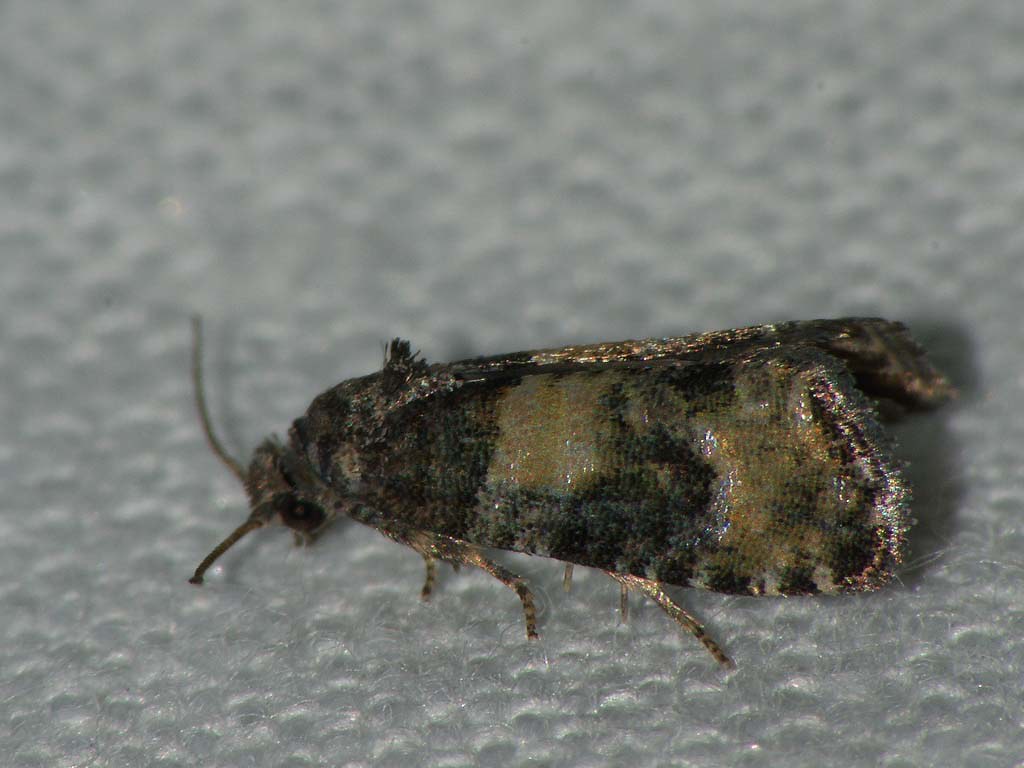This close-up photo showcases what appears to be a moth, perched on a textured white fabric surface, possibly a rug or napkin. The moth's wings, predominantly black and gold, shimmer under the light, with the golden areas particularly catching the eye. These wings possess a mix of grayish and greenish hues, and wide, opaque stripes. The moth's fuzzy head features one noticeably shorter antenna, which may have broken off. Its face is angled downward, revealing one large black eye. The moth's legs are golden, marked with alternating black and gold stripes, and three legs are visible on one side. Despite its striking colors, the moth appears unhealthy or possibly dead, with patches of what looks like yellowish fungus or pus on its wings. The background, a slightly out-of-focus bubbled texture, contrasts with the detailed, vivid depiction of the moth.